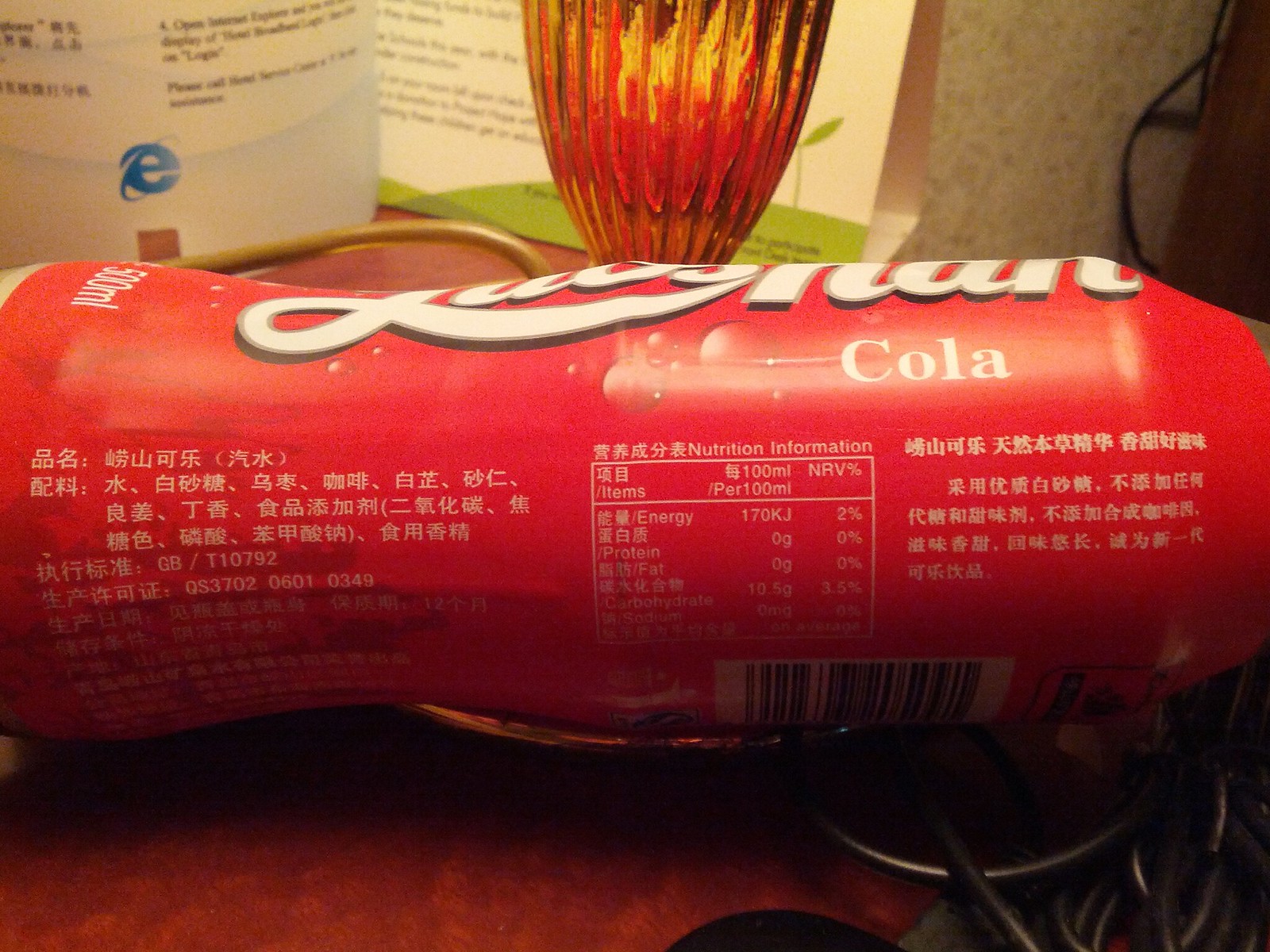This is a close-up color photograph of a horizontally placed Coca-Cola bottle on a table. The table surface, visible at the bottom of the image, showcases a beautiful hardwood finish. Just beneath the bottle, a few metal rings can be seen, adding an interesting texture to the composition. The bottle, intended for either the Chinese or Japanese market, displays characters in one of these languages. This side of the bottle features nutritional information and ingredients, all written in the respective language. The very tip of the bottle's front is partially visible, with the word "Cola" in English and a fragment of the iconic Coca-Cola logo peeking through.